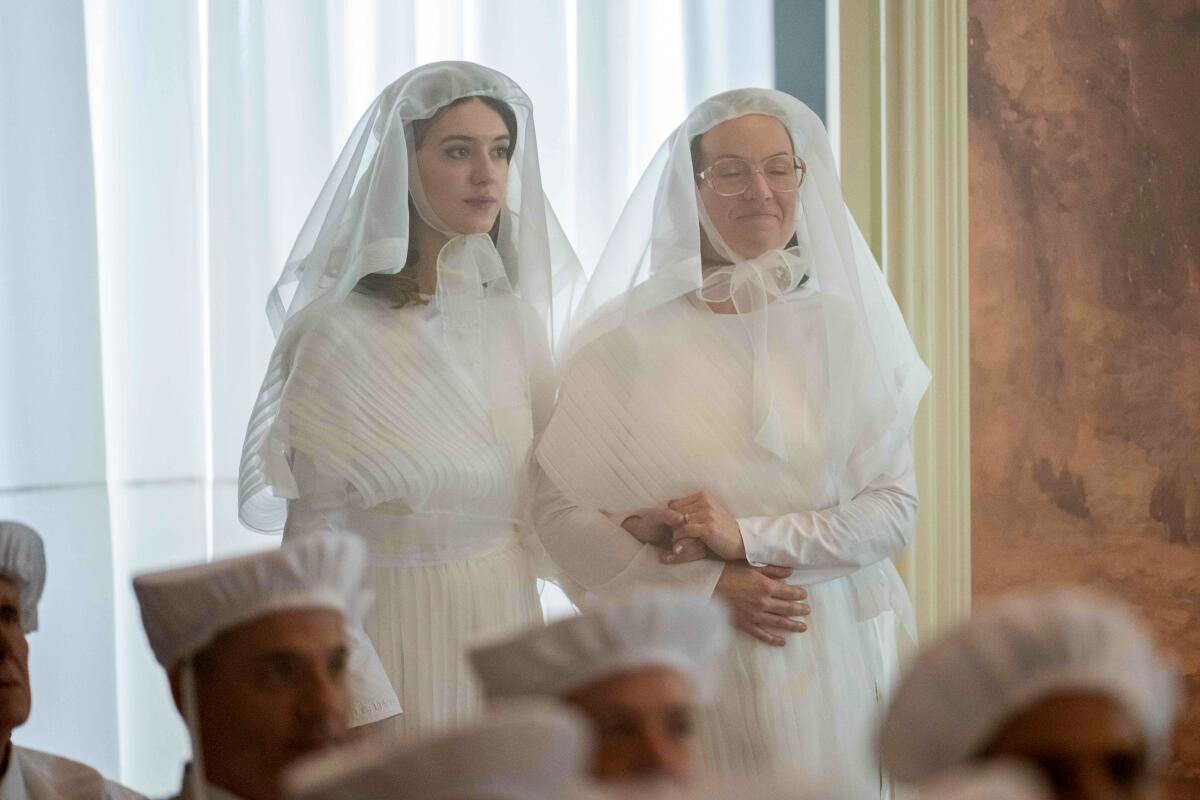This colored photograph, taken indoors, features two white women standing in what appears to be a church or some other ceremonial setting. At the center, they are dressed in white gauzy dresses and have sheer white scarves tied in bows under their chins, resembling headdresses. The older woman on the right, likely in her mid to late 40s, wears glasses, has her eyes closed, and a subtle smile. The younger woman on the left, probably in her early 20s, has her eyes open, staring intently forward, wearing makeup, and they are holding hands, suggesting a comforting or supportive gesture, possibly between a mother and daughter. Behind them, a large window draped with a sheer curtain dominates the background, and a partial view of a brown wall is visible on the right edge. In the foreground, several men are seated, wearing white caps or bonnets, though their faces are blurred. The scene suggests a significant event, perhaps a wedding or religious ceremony, set within a close-knit community, possibly Amish. Neither woman is adorned with any jewelry, emphasizing a simple, humble aesthetic.